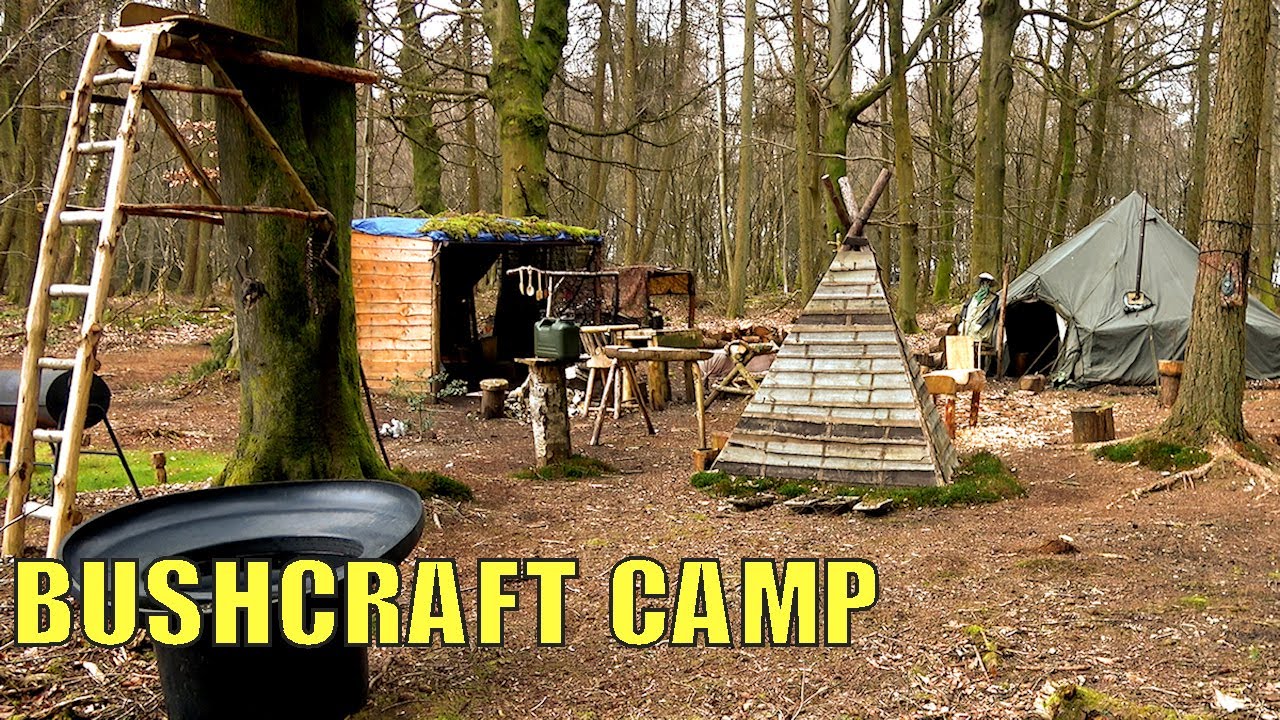The image depicts a rustic campsite located in the middle of a dense, leafless forest. At the bottom left of the image, the words "Bushcraft Camp" are prominently displayed in large yellow font. Dominating the center of the campsite is a makeshift wooden teepee, constructed in a triangular shape with sticks protruding from the top. To the right of the teepee is a traditional camping-style tent of gray or olive green color, appearing slightly more modern amidst the rustic setup. In front of the tent, a figure with a white hat and matching poncho can be seen, though their back is turned to the camera, making their features indistinguishable.

On the left side of the campsite, a tall ladder made from light-colored wood leans against a large tree trunk, leading up to a rudimentary wooden platform likely used for elevated vantage, possibly for hunting. Nearby, there is a wooden enclosure covered with a blue tarp, which appears weighted down and might be used for storage or cooking. Scattered throughout the campsite are various wooden items, along with some circular device that could potentially be a rain-catching apparatus. The ground is primarily dirty, with twigs, patches of grass, and weeds interspersed among the brown dirt and wood chips. The barren, mossy trees encircle the campsite, contributing to the sense of an untouched natural environment in what seems to be the winter season. No other people are visible in the scene, emphasizing the solitude of this forest encampment.